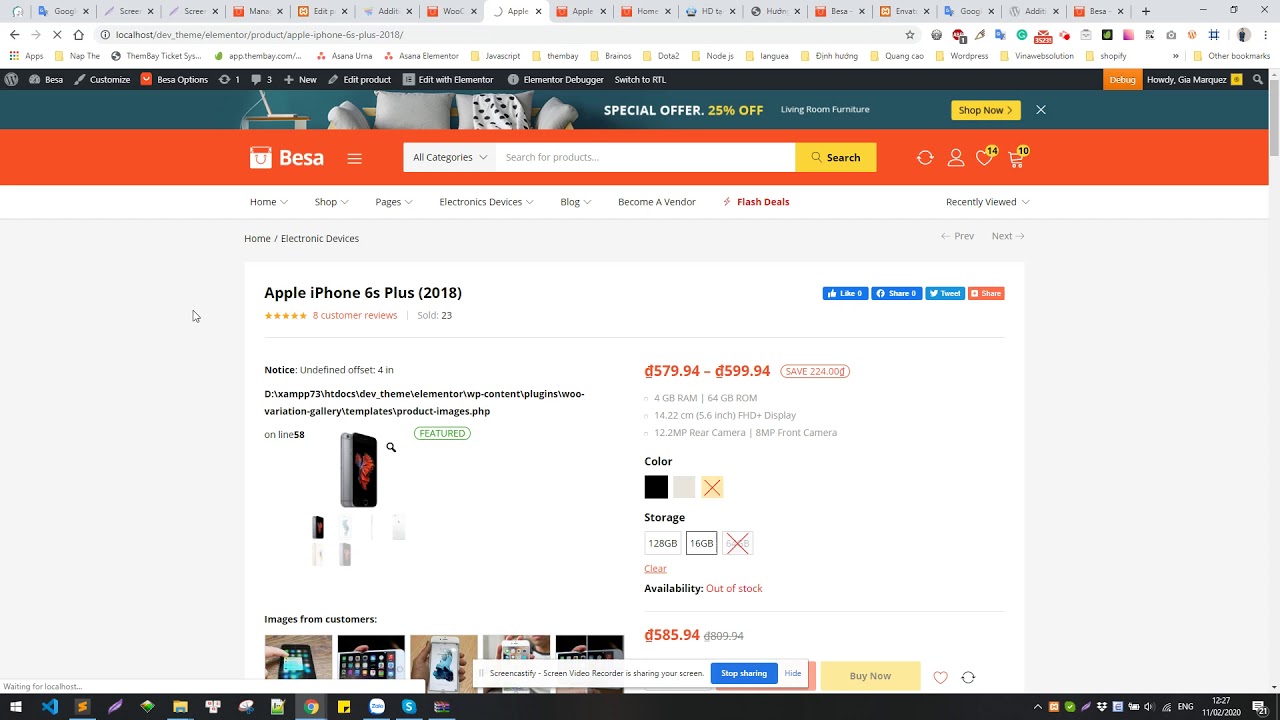A detailed and cleaned-up caption:

This is a screenshot of the BESA.com website displayed in a web browser on a computer. The browser is cluttered with numerous open tabs, with the BESA page being the seventh one from the left and currently in focus. At the very top of the BESA page, there's a prominent blue banner announcing a "Special Offer: 25% Off" on living room furniture, with an image of a couch to the left and the promotional text to the right. The banner also includes a "Shop Now" button in a yellow box situated towards the right, followed by a small "X" icon for closing the banner. Below this is the website's header, distinguished by its orange color. On the left side of the header is the BESA logo, and to the right of it is a menu icon. Centrally placed within the header is the search bar featuring a drop-down menu for selecting "All Categories" on the left, and a yellow search field on the right. The main body of the webpage, set against a white background, displays information about an Apple iPhone 6 Plus, including various thumbnails, price details, and additional product information.